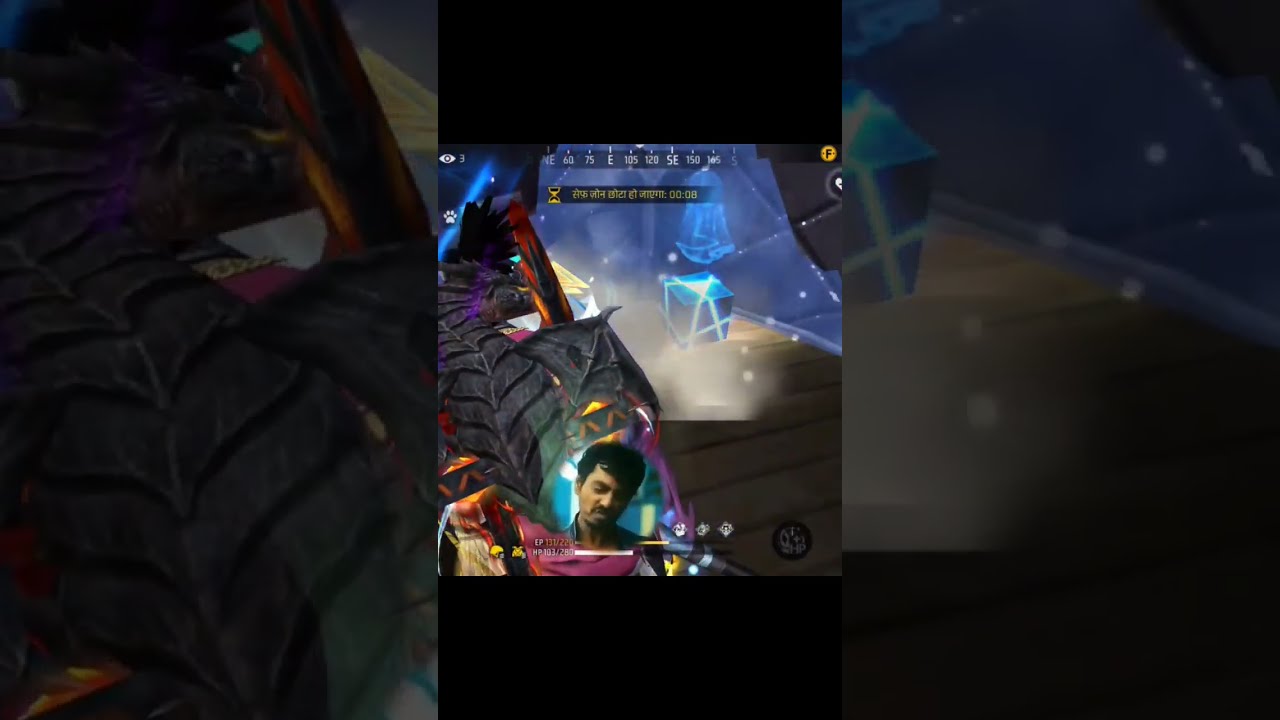The image appears to be a complex and surreal mashup that seems to depict a scene from a computer-generated environment, possibly a video game. Dominating the left side is what looks like tire tread or possibly an armored exoskeleton with an orange glow, while the right side features white smudgy dots. Central to the image is the head of an Indian man, rendered in shadow, with his face partially visible and slightly sneering, placed towards the bottom of the frame. Above his head is a set of directional compass numbers with an 'E' for East, suggesting a navigation element commonly found in games.

In the background, there's a glowing turquoise-blue chest or cube with yellow banding, which creates the impression of containing something valuable like treasure or superpowers. The scene is set in what resembles a room with a wooden-paneled floor. The entire image is vertically oriented and bordered by blown-up, indecipherable close-ups of the same scene on either side, giving it a surreal depth. The overall effect is a chaotic mix of visual elements, evoking a sense of bewilderment and intrigue.